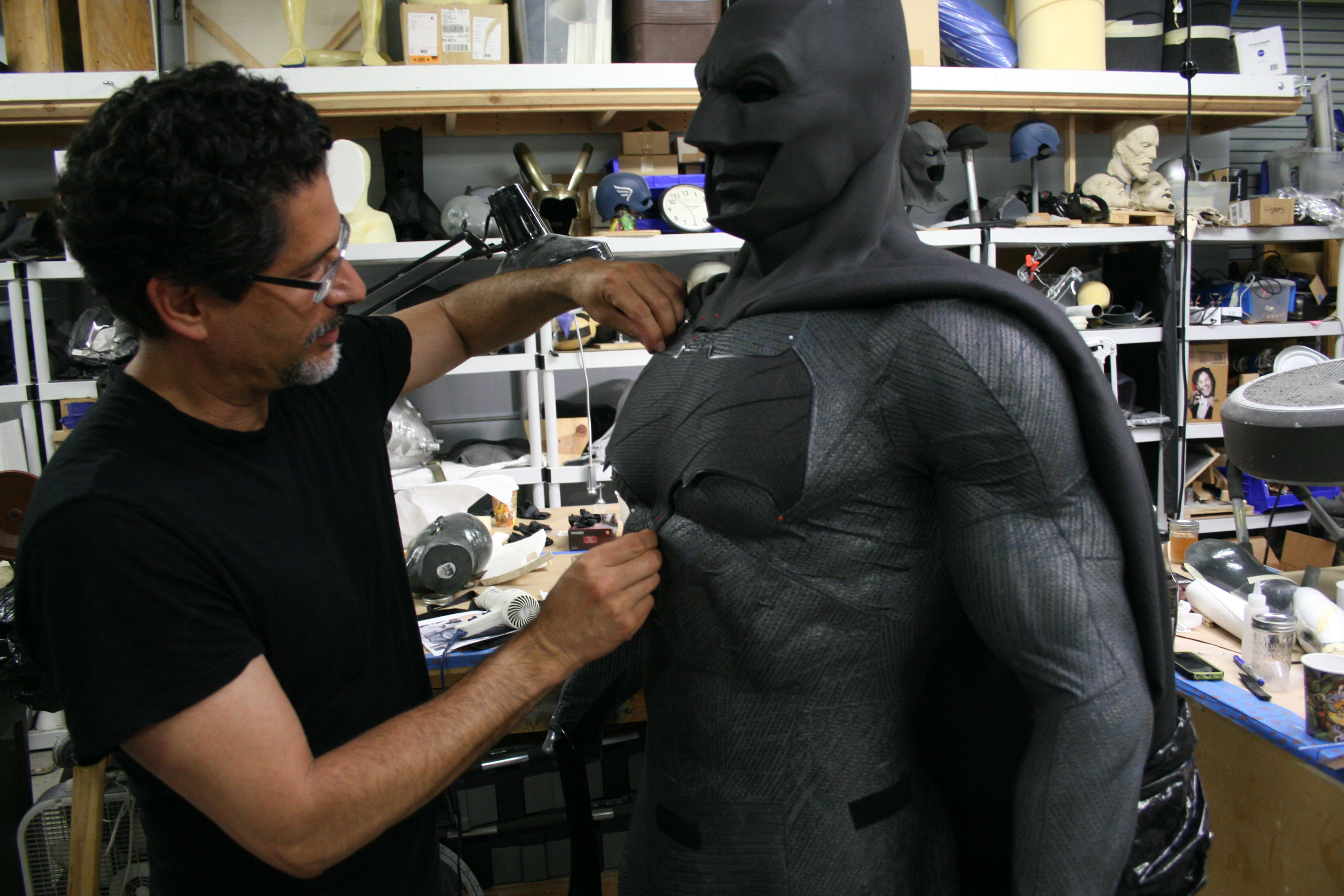A horizontally aligned rectangular photograph features a middle-aged Hispanic man with black hair, styled just past his ears in a bushy or curly manner, and salt-and-pepper facial hair, including a gray beard and a small goatee. He is wearing black-rimmed glasses and a short-sleeved black t-shirt. The man stands in what appears to be a cluttered workshop or store, with numerous shelves and desks packed with a variety of items such as busts, boxes, and various unidentifiable objects.

In the photograph, the man is intently focused on a black Batman costume he appears to be adjusting. His hands are positioned on the chest area of the costume, which features a gray patch. The Batman figure has a face mask, a cape, and massive biceps, creating an imposing presence. It is unclear whether the costume is worn by a person or is simply a statue. The background showcases the crowded workspace, filled with numerous objects including another bust, a possible radio, tubes, jars, and even what seems to be a wheel in the lower right corner. The detailed and densely packed scene reflects the intricate and dedicated work involved in crafting or adjusting the Batman figure.